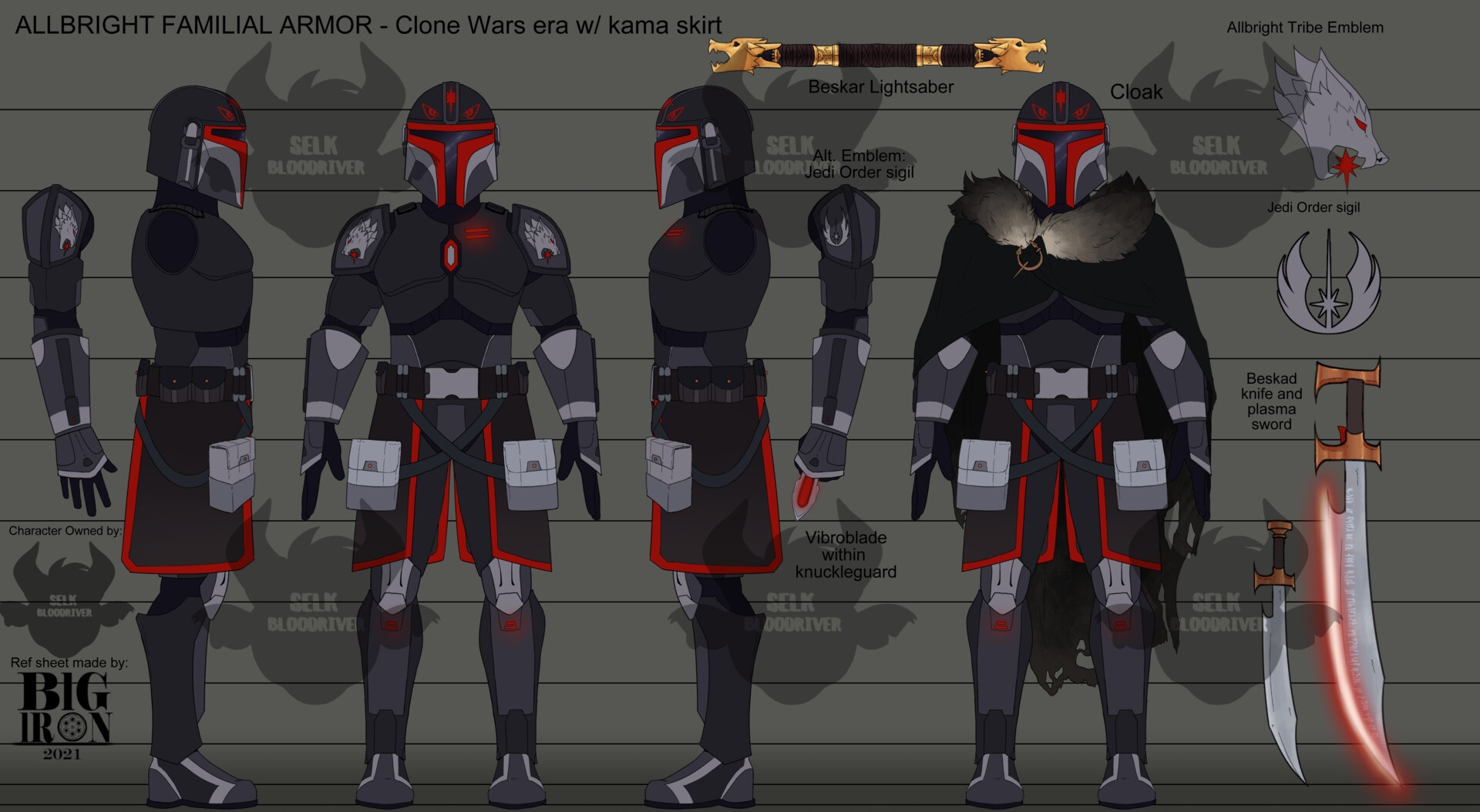This image is a detailed cartoon-style representation of a Clone Wars-era figure titled "Albright Familial Armor" with a kama skirt. The main focus is a character depicted in different stances: facing right, forward, left, and again forward but fully garbed, showcasing multiple views of the armor. The armor is predominantly black with gray and red accents, including a red trim on the helmet and red highlights on the attire. Specific elements include a black belt with a gray buckle, a plaited skirt, and a distinctive animal pelt-style coat featuring a fur collar.

The armor ensemble also includes practical elements like holsters and satchels on the front, and various weapons such as a machete, a sword with a laser-like feature, and several standard blades are depicted. The intricate design shows influences from Mandalorian aesthetics, comparable to Boba Fett's armor, with some suggesting the figure might be a Republic soldier or a bounty hunter.

The background of the image contains watermarked drawings, specifically a logo in the lower-left corner which resembles the head of a boar or bull and reads "Made by Big Iron, 2021."